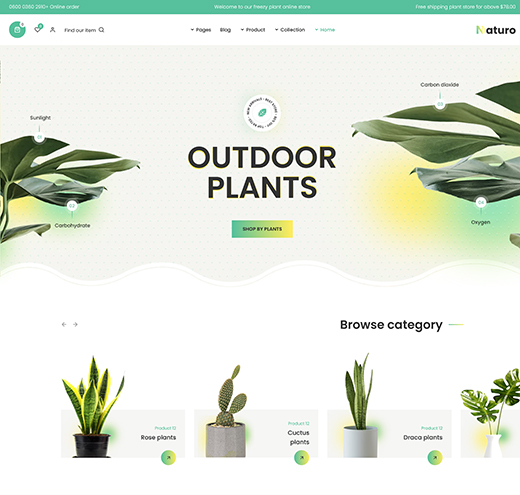Here is a cleaned up and detailed caption for the image described:

---

This image is a screenshot of the homepage of a website named "Naturo." In the top left corner, the Naturo logo is prominently displayed, with the letter "N" featuring a gradient of green and yellow, while the remaining letters are bold and black. Below the logo is a detailed illustration of a leaf, with its different parts labeled in small black print.

Dominating the center of the page is a large, bold, black title that reads "OUTDOOR PLANTS." Directly beneath this title, there is a gradient bar that transitions from green on the left to yellow on the right, with the words "Shop by Plants" displayed prominently.

Toward the bottom of the page on the right side, the text "BROWSE CATEGORY" is shown in large, bold, black letters. Underneath this heading, there are five thumbnails, each depicting a different potted houseplant. The name of each plant is listed to the right of its respective thumbnail, accompanied by a small gradient button that likely serves as a purchase link.

---